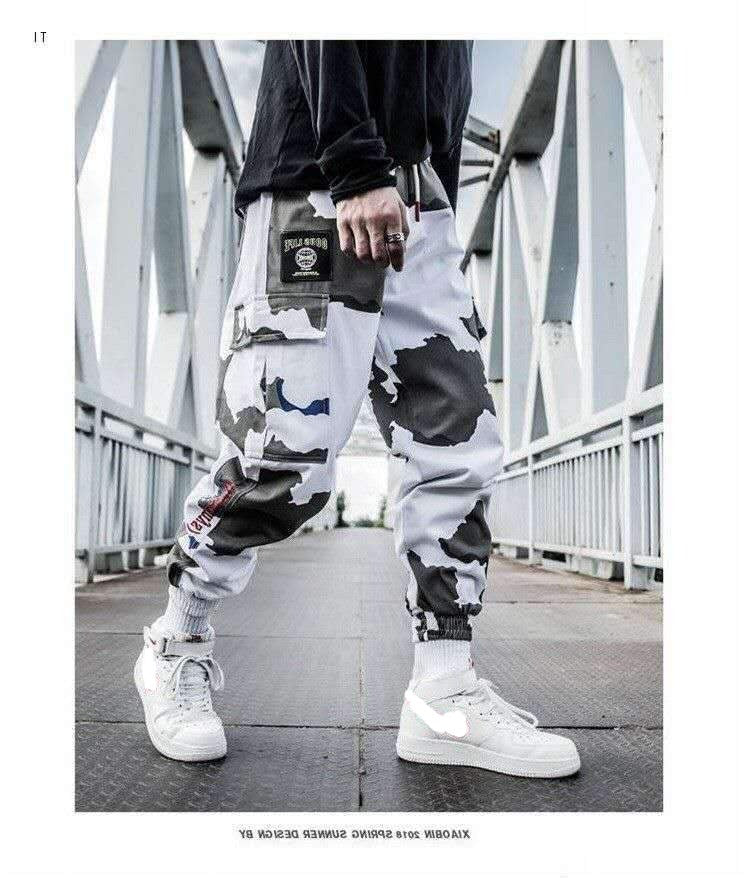This realistic-looking vertical photograph captures a scene of a man standing at the center of a white metal pedestrian bridge. The structure's sides—composed of a crisscross pattern of metal grating—rise approximately 20 feet, with hand railings running along both edges. The bridge's floor is made of solid black corrugated metal, with distinct seams visible. The man, observed from around the chest down to his feet, is dressed in a long-sleeve black shirt and white-and-black camouflage-style pants. His footwear includes distinctive white lace-up sneakers with metallic swooshes, white athletic socks, and an additional Velcro strap at the top of each shoe. On his right hand, he wears a ring on the index finger. His pants bear an unreadable brand label near the pockets. The background of the image features a light blue daytime sky, with hints of greenery and white elements at the far end of the bridge. Text reading "IT" appears in black font on a white background in the top left corner of the photograph, while more difficult-to-decipher black text is visible along the bottom.